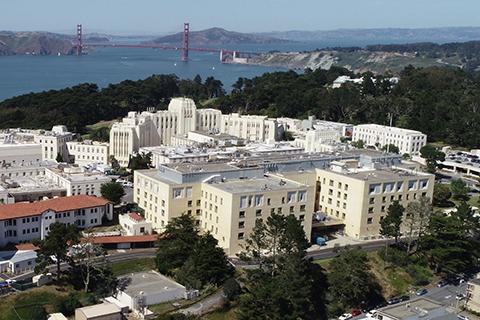This aerial photograph captures a suburban area that could be mistaken for San Francisco, given the resemblance of the suspension bridge in the background to the Golden Gate Bridge. The main focus is a cluster of interconnected white buildings, predominantly five to six stories high, with square windows. Adjacent to these, on the left, is a contrasting three-story building sporting a red roof, likely a motel, and a single-story structure with a matching roof in front of it. The scene is rich with greenery, as trees envelop the buildings, which sit near a sizable waterway flowing from the upper left to the upper right of the image. The background features a range of low hills under a murky blue-gray sky, enhancing the suburban feel of the landscape. Distinct roads and scattered cars add to the serene, yet populated, atmosphere of this picturesque locale.